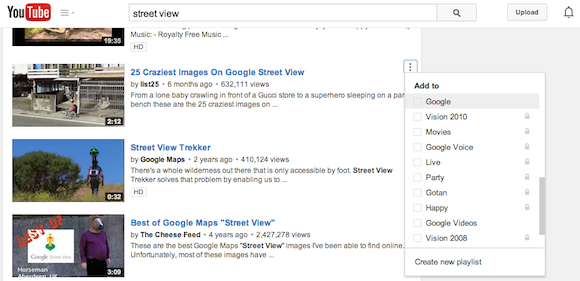**Detailed Caption:**

This image is a screenshot of a YouTube desktop page. In the top left corner, the YouTube logo is prominently displayed, featuring a black "You" and a white "Tube" enclosed within a red box. The search bar contains the text "street view," with an adjacent search icon, an upload button, and a notification bell.

The search results begin with a video titled "25 Craziest Images on Google Street View," visible through its thumbnail, which shows a snippet with a duration of 2 minutes and 12 seconds. Below this, another video titled "Street View Trekker by Google Maps" shows that it was uploaded two years ago and has garnered 410,124 views. The thumbnail for this video features a bush with a blue sky in the background and a robot-like figure on the left.

The final video in the search results is titled "Best of Google Maps Street View" by TheCheeseFeed and was uploaded four years ago. This video has accumulated 2,427,278 views. The thumbnail displays a man standing with the text "Best of Best of" and "Google Street View."

To the right of these search results, the user has clicked on the three vertical dots, opening a context menu. This menu lists options such as "Add to," with several playlists underneath, including "Google," "Vision 2010," "Movies," "Google Voice," "Live," "Party," "GoTen," "Happy," "Google Videos," "Vision 2008," and an option to "Create New Playlist."